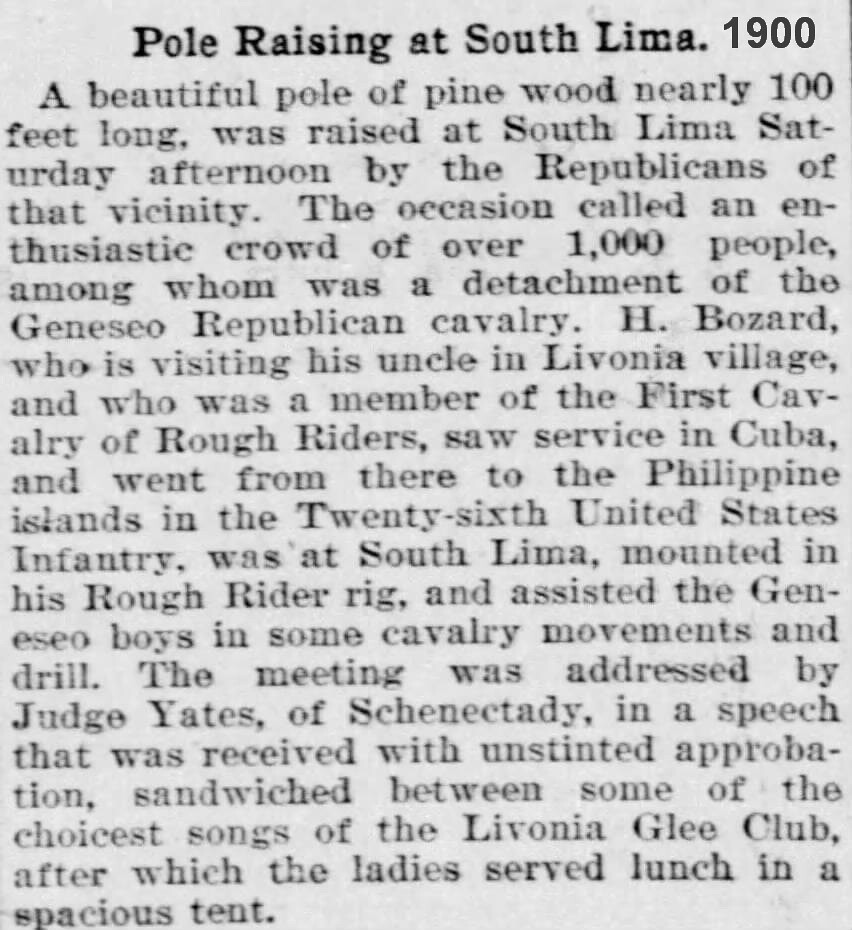**Pole Raising at South Lima, 1900**

A beautiful pinewood pole, nearly 100 feet long, was raised at South Lima on Saturday afternoon by the local Republicans. The event drew an enthusiastic crowd of over 1,000 people, including a detachment of the Genozo-Republican Cavalry. Among the attendees was H. Basel (or H. Bouzard), who had been visiting his uncle in a nearby village and had distinguished service history. As a member of the First Cavalry of Rough Riders, Basel had seen action in Cuba and later served in the 26th United States Infantry in the Philippine Islands. Mounted in his Rough Rider attire, he participated in cavalry movements and drills with the Genozo Boys. The assembly was also addressed by Judge Leitz, adding to the day's significance. After the pole raising, lunch was served in a spacious tent, rounding off a memorable afternoon. The gray-toned image, with its black printed text, appears to be a clipping from either a newspaper or book, marked by the bold title "Pole Raising at South Lima, 1900" prominently displayed at the top.